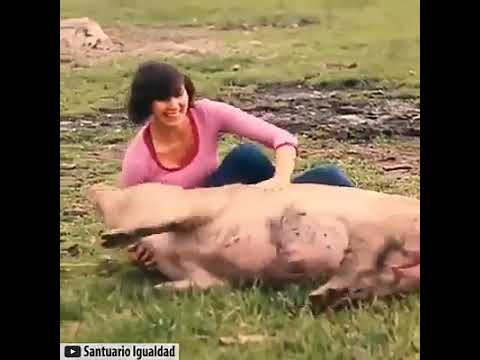In this interesting and somewhat blurred image, a woman with dark short hair is lying on the grass, smiling and enjoying herself as she interacts with a large, pinkish-gray pig. The woman, dressed in a pink long-sleeve blouse with red trim and blue jeans, has one hand scratching the pig and the other nestled under its neck. The pig appears relaxed and content, lying on its side with one front leg raised. Behind them, a visibly muddy and wet area can be seen with some exposed rock. Both seem to be having a good time in this outdoor, grassy setting. At the bottom left of the image, the text “Santuario Igualdad” is visible, along with thin vertical black bars on either side, indicating that the image may have been sourced from YouTube.